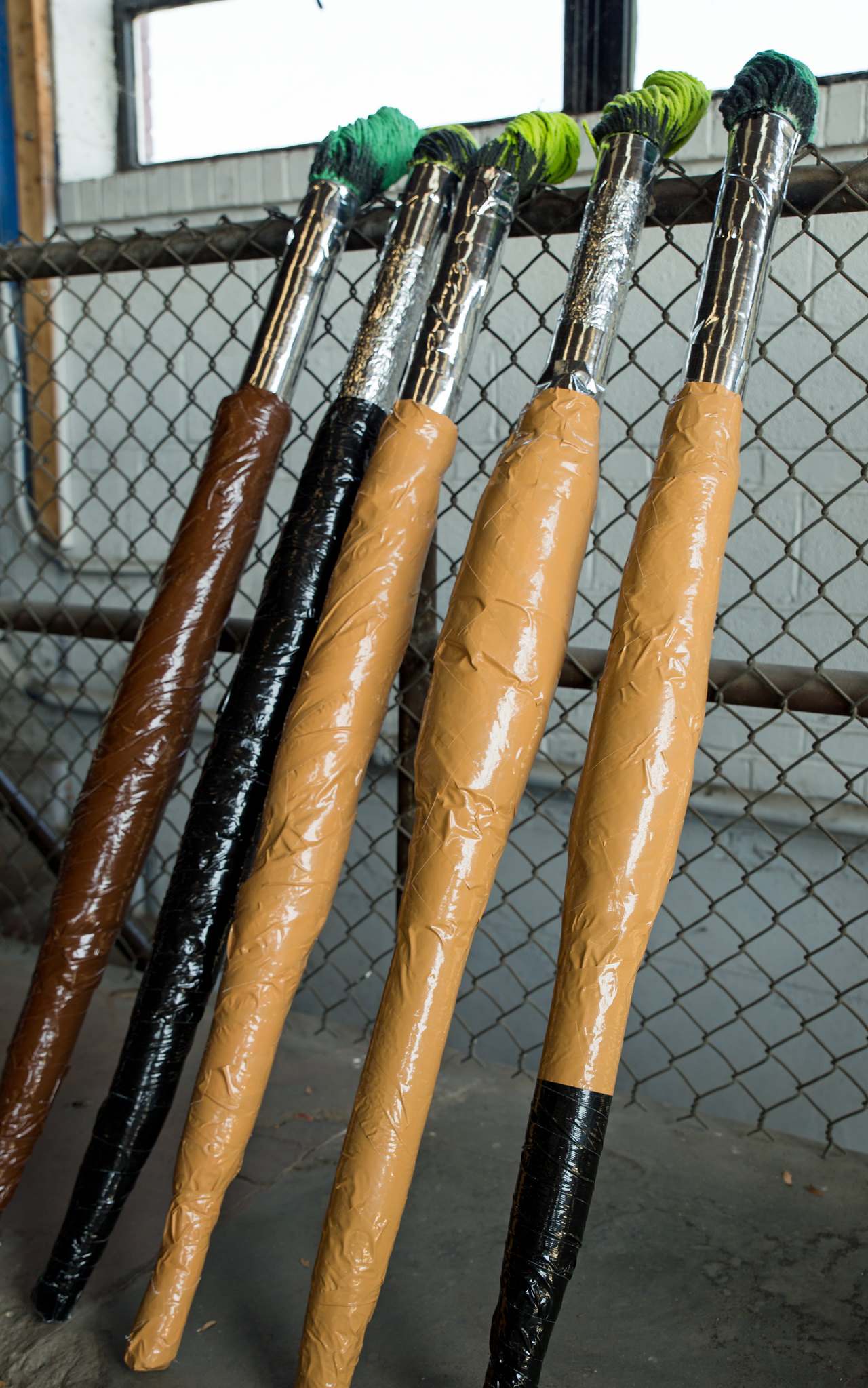This photo features five oversized, paintbrush-like sculptures leaning against a dark gray chain-link fence. The elongated handles, occupying almost the entire frame and measuring approximately 16 inches, are wrapped in various shades and textures of shiny tape. From left to right, the first paintbrush-like object is wrapped in dark brown tape, the second in black tape, the next two in a light tan tape, and the final one combines tan tape with a black tip. Each handle transitions into a silver section, resembling the ferrule of a paintbrush, which ends in tightly wrapped green yarn or paint, suggesting the bristles. The setting includes a white brick wall visible through the gaps in the fence, and they rest on a cement floor. The intricate details and varied materials lend a unique, almost sculptural quality to these large-scale replicas.